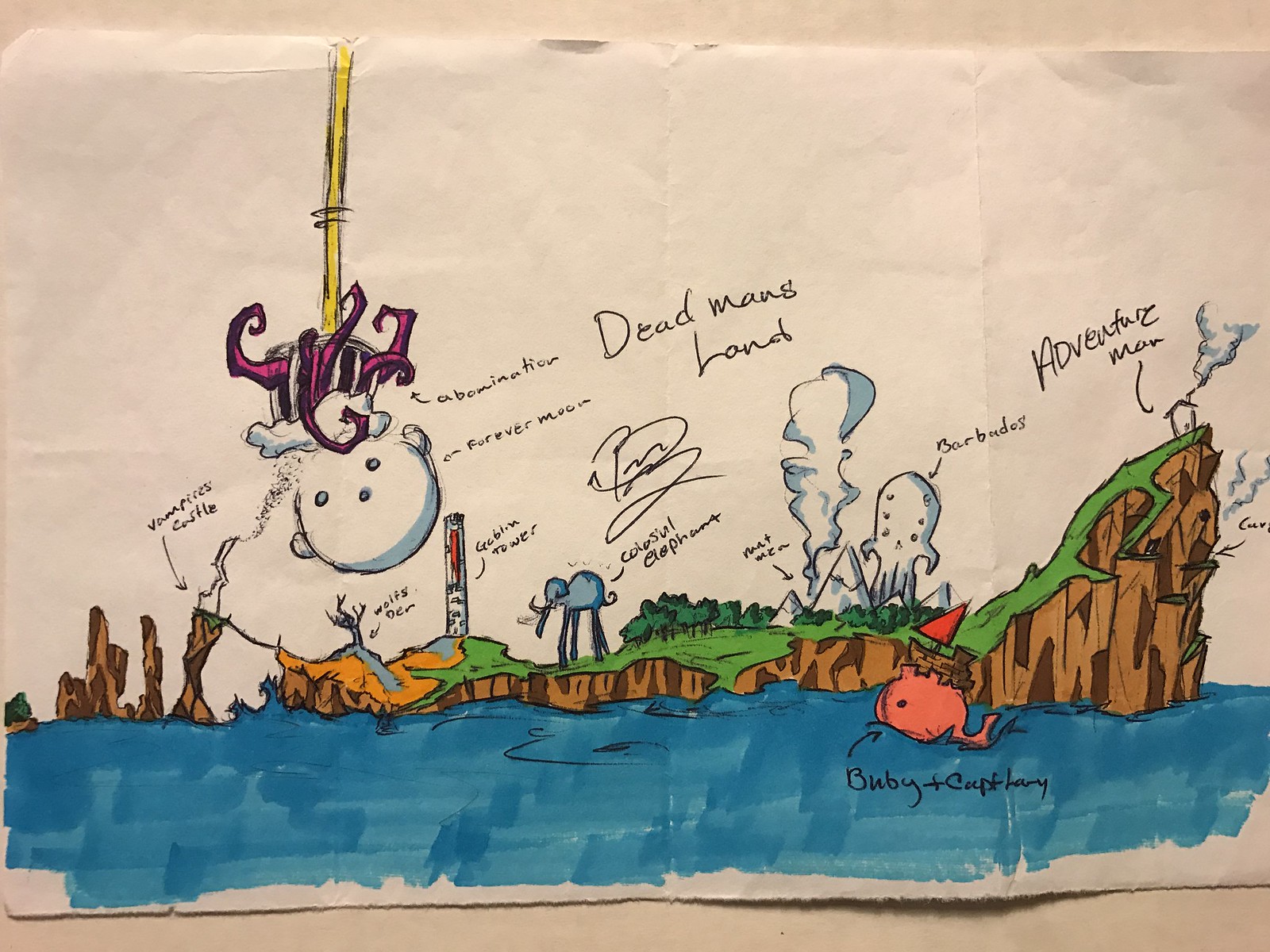The image appears to be a surreal, detailed drawing or painting potentially intended as a preliminary sketch for a larger mural or artwork. It features a richly diverse landscape with several distinct areas. 

In the bottom section, there's a body of water, likely a river, with various labeled creatures both in and around it, including a whale and a colossal elephant with unusually long legs. Above the water lies a small rocky island with grassy terrain and some trees. This island is dubbed "Dead Man's Land," a title prominently inscribed in the center of the image. The landscape includes multiple regions: hilly grasslands where an "adventure man" stands, a forest adjacent to a mountain, and a desert on the far left.

Dominating parts of the scene are several unusual and whimsical elements. A yellow, pipe-like object descends from the top left, featuring a claw-like appendage that holds a pink, octopus-like creature. Nearby, there's a white, balloon-shaped figure with eyes, a nose, and ears but no mouth, floating mysteriously. Accompanying these are a tower, a boat, a spiky outcrop, and a clay-like rock formation labeled with various titles in ink.

Additional fantastical features include a forested area with a tentacled figure resembling a squid, and a Coliseum-like structure emanating more tentacles. The terms "abomination, forever moon, vampire's castle," and "Barbados" are among the various labels that dot the landscape, each next to their corresponding feature, creating a whimsical, annotated map-like quality. This vividly imaginative scene conjures a mythical place full of adventure and oddities.